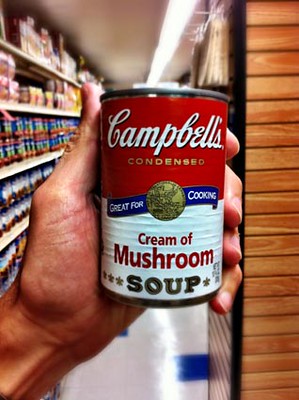A Caucasian male hand is prominently holding a metal can of Campbell's Cream of Mushroom soup. The can features a distinctive design with a red upper section and a white lower section. The brand name “Campbell's” is written in elegant white script across the red part of the label. Below it, the word "Condensed" appears in gold. Further down, a blue banner with white text reads "Great for Cooking," and beneath that, "Cream of Mushroom" is displayed in bold red text, with "Soup" at the very bottom in a combination of gold and black text.

In the background, the upper left area is filled with numerous grocery store shelves, well-stocked with various other cans of soup and different brands. The ceiling is an understated off-tan color, fitted with a row of fluorescent lights that illuminate the setting. On the far right side of the image, a subtle wooden support column made from light blonde wood adds to the structural integrity of the space. The detailed yet ordinary supermarket scene offers a slice of everyday life, focused on a staple item in many households.